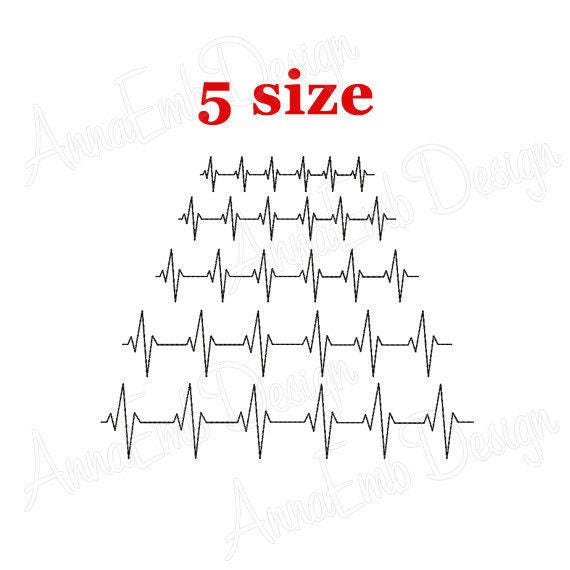This diagram illustrates five zigzag lines, resembling those seen on a heart rate monitor. These lines display a consistent pattern across each row: a peak at the top, a drop to the bottom, a rise back up, a slight descent, and then a horizontal stretch. This sequence repeats six times per line. The lines are arranged in descending order of length, with the longest line at the bottom and each subsequent line progressively shorter, culminating in the shortest line at the top. Above these lines, red text reads "five size" against a white background adorned with cursive script.